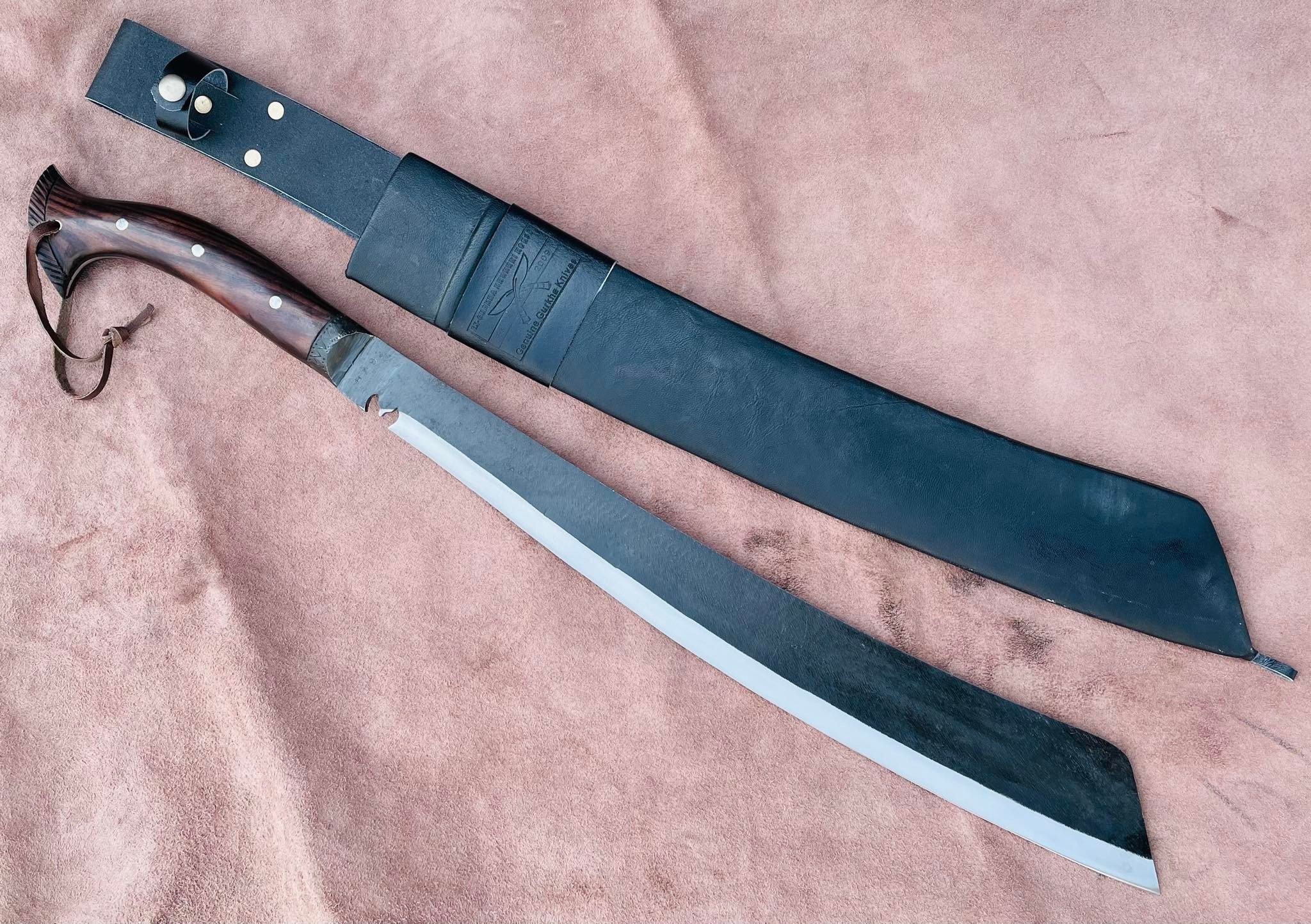This detailed photograph showcases a unique machete-type sword and its accompanying leather sheath, both arranged on an elegant pinkish suede cloth. The sword, approximately three feet long, features a meticulously carved eagle's wings near the base of its blade, adding an artistic touch to its formidable design. The wooden handle, gently curved and beautifully crafted, is secured with three golden screws and includes a thin leather tie threaded through a hole at its flared end. The blade itself is mostly straight with a slight upward curve, expertly beveled and sharpened, resembling a Viking's sax. Notably, there's a notch in the blade near the handle, pointing to both its functional and aesthetic intricacies. The sword's sheath, made of thick leather, has a belt attachment and an embossed design—either an eagle or crossed knives logo—which adds to its rugged elegance. Both items are finely presented on the suede cloth, with the handle of the sword positioned towards the left, highlighting the craftsmanship and detailed artistry involved in both the weapon and its protective case.